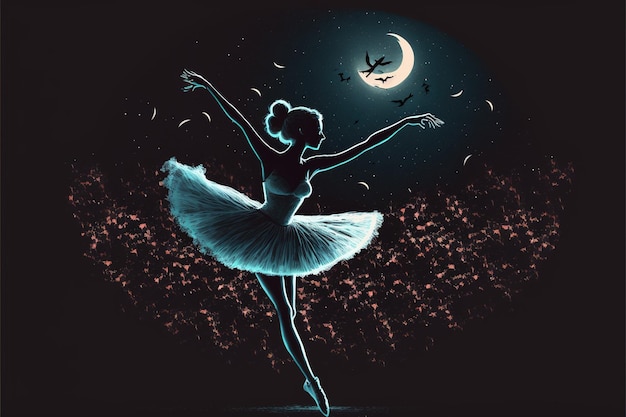This is a detailed digital illustration of a ballerina against a moonlit, nighttime sky. The backdrop predominantly features a black, oval-framed night scene with a dark blue tint. A bright, crescent moon occupies an off-center position in the sky, flanked by the silhouettes of tiny birds or bats flying before it. Scattered across the sky are white specks, possibly representing stars, or feathers, or giving an ethereal fairy dust effect.

In the foreground, the ballerina is positioned gracefully on pointe, her body outlined with bright moonlight while her details remain in shadow. She is dressed in a traditional light-colored or powder blue tutu that billows out around her waist. Her hair is neatly styled in a bun, and her arms are extended delicately to either side, giving an appearance of elegance and poise. The ballerina faces to the right, with her right leg supporting her weight and her left leg raised, visible only from the top.

Surrounding the ballerina are what seem to be cherry blossom petals, reddish-orange speckles, or possibly flower petals she is tossing from her fingertips into the air, adding a dynamic, whimsical element to the scene. Overall, the image combines the serenity of a moonlit night with the grace and fluidity of ballet, creating a captivating and serene visual narrative.